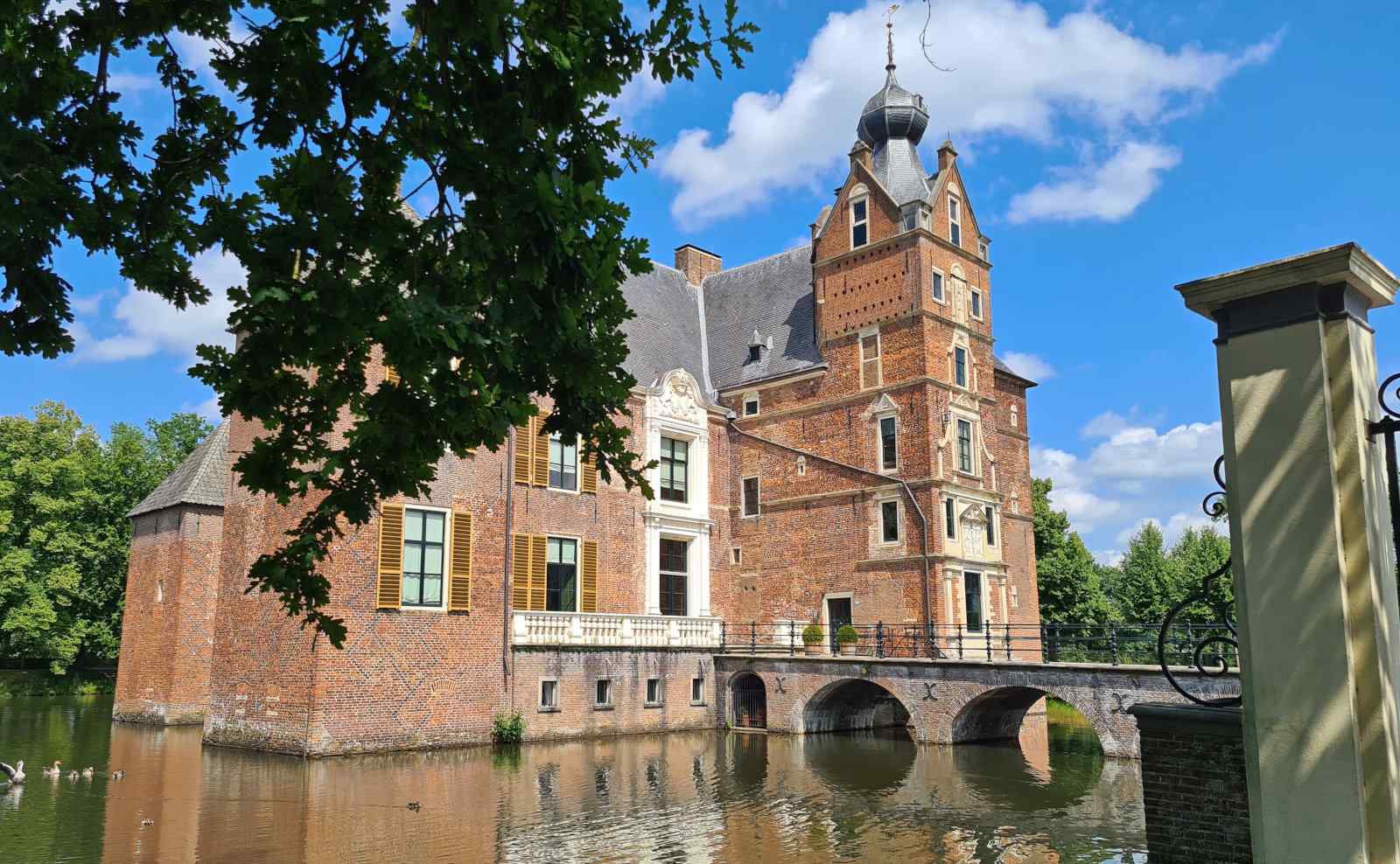This picturesque scene features a large, historic, reddish-brown brick building that resembles a castle, complete with a tall tower and a chimney on the right. Set atop a body of water, the structure's base shows signs of being worn and faded from constant contact with the water. A charming bridge with railings, intended for pedestrians, extends from the land to the entrance of this imposing building. Beneath the bridge, two semicircular channels allow water to flow through. The building, adorned with yellow and white siding on some windows, and shutters indicating it is well-maintained, has a prominent section rising higher than the rest, crowned with a dome. In the tranquil water below, ripples dance as a family of ducks or geese swims nearby, along with another bird of a different kind. The background is lush with trees under a brilliant blue sky, dotted with a few clouds, enhancing the serene and timeless beauty of the scene.